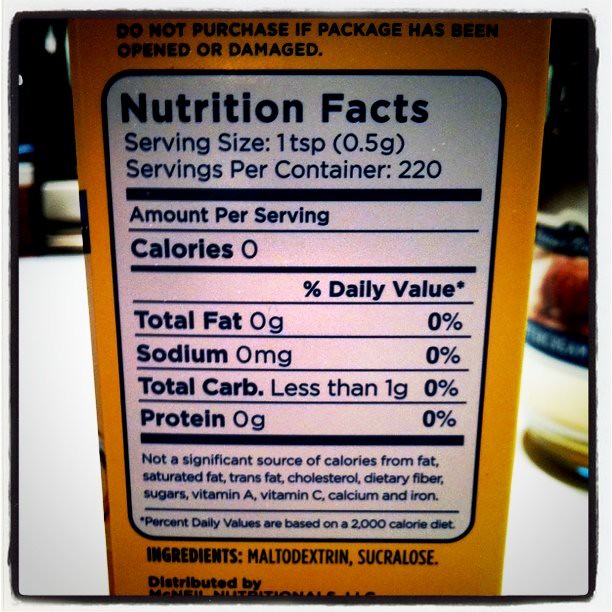The photograph shows the side panel of a yellow food carton with a detailed view of its nutrition facts label and additional elements in the background. The top of the carton features a warning in black font: "Do not purchase if package has been opened or damaged." Centrally placed within the yellow box is a white rectangular section bordered in black, containing the nutrition facts. The label lists a serving size of one teaspoon (0.5 grams) and highlights that the container holds 220 servings, each with zero calories. Key nutritional values are noted as well: total fat zero grams (0%), sodium zero milligrams (0%), total carbohydrates less than one gram (0%), and protein zero grams (0%). The ingredient list includes maltodextrin and sucrose. Below the nutrition facts, distributed by information extends off the bottom of the image.

Surrounding the carton, on the left and right sides, are white tables extending about two-thirds up the page, against a predominantly black backdrop. On the left side, toward the top, there is a visible white chair and a small square shape originating from the left edge of the frame. Just to the side of the carton, partially off-screen, there appears to be an apple on a blue plate, along with a yellow banana peeking into the frame from the bottom.